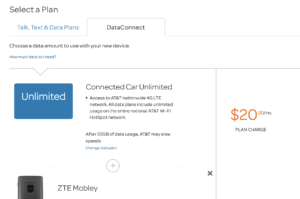This low-resolution image, cropped and hard to distinguish, appears to display information about a data plan, potentially for a car or mobile service. The background is predominantly white with a title indicating "Selected Plan." The main header "Talk, Text, and Data Plans" is highlighted in blue. A secondary tab labeled "Data Connect" is outlined in gray text, suggesting this is the current selection. Underneath, there is some legible text followed by a bullet point within a blue and white box that reads "Unlimited and Connected Car Unlimited," though the detailed bullet point description is illegible. A blue hyperlink is visible below this section. To the right, written in orange text, are the details "$20/MO, 20 month plan change," and underneath it, references "CTE Mobily X." An indiscernible dark gray icon is also present. Despite the image’s poor quality, it seems to pertain to selecting or managing a car-related mobile data plan.